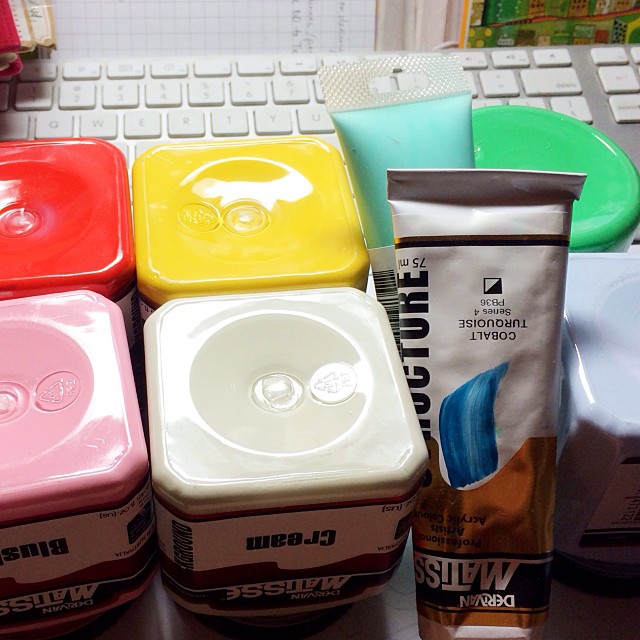The image shows a collection of various containers and tubes, primarily aligned in an upside-down orientation on a desk. The containers resemble paint bottles or perhaps muscle-building supplements, each labeled with different colors and partially visible text. Notably, one white container has blue letters that spell out "cream," and another light pink container might read "blush," though the text is partially cut off. There are also distinctly colored containers: one with a pink base, another with a yellow base, and one with a red base. Additionally, tubes of paint are visible, including one with a white label and black text that reads "cobalt turquoise." Another tube seems to be turquoise with an illegible label except for part of the barcode, indicating it is a different brand. To the right, a pale lilac-colored bottle and a circular green jar are present. In the background, a gray and white keyboard is partially visible, accompanied by what appears to be a piece of paper with writing on it running along the wall.